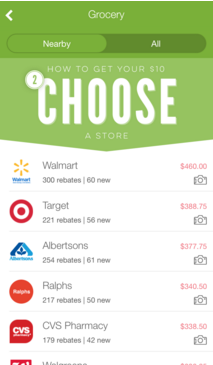This screenshot from an unspecified app features a predominantly green header section indicating "Grocery Nearby," which is currently selected. Below this, the app displays a list of stores along with their rebate details: Walmart offers 300 rebates, including 60 new ones, totaling $460; Target provides 221 rebates, with 56 new, amounting to $388.75; Albertsons lists 254 rebates, including 61 new, worth $377.75; Ralphs features 217 rebates, 50 of which are new, summing up to $340.50; CVS Pharmacy has 179 rebates, 42 new, totaling $338.50. The partially visible name "Walgreens" is cut off at the bottom edge of the vertically-oriented image. The screenshot contains only text and lacks any photographic elements or visuals such as people, animals, plants, automobiles, or airplanes.